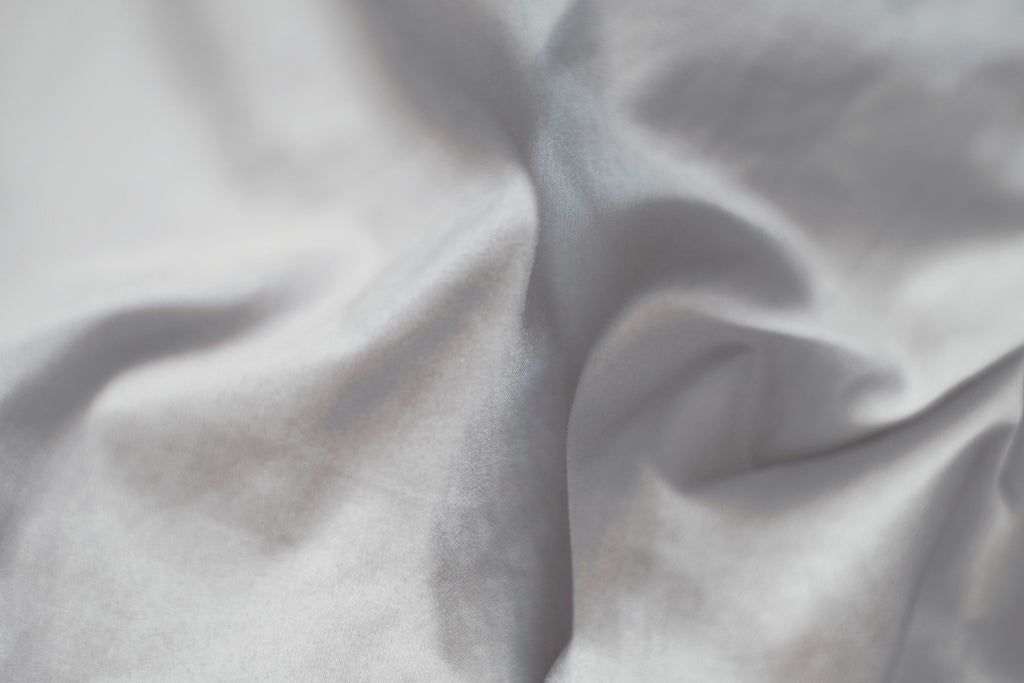This close-up image captures a crumpled, white fabric, intricately arranged to emphasize its textured folds and shadowed creases. The fabric, likely cotton or satin due to its subtle shine, appears almost sculpted, with shadows in gray tones accentuating its curves and wrinkles. The photograph uses medium-level natural lighting, making it difficult to determine the setting. The high-quality cloth, possibly linen, features a blue-white hue, and the overall scene maintains a simple, minimalistic approach, focusing solely on the fabric's intricate details and soft, woven nature.